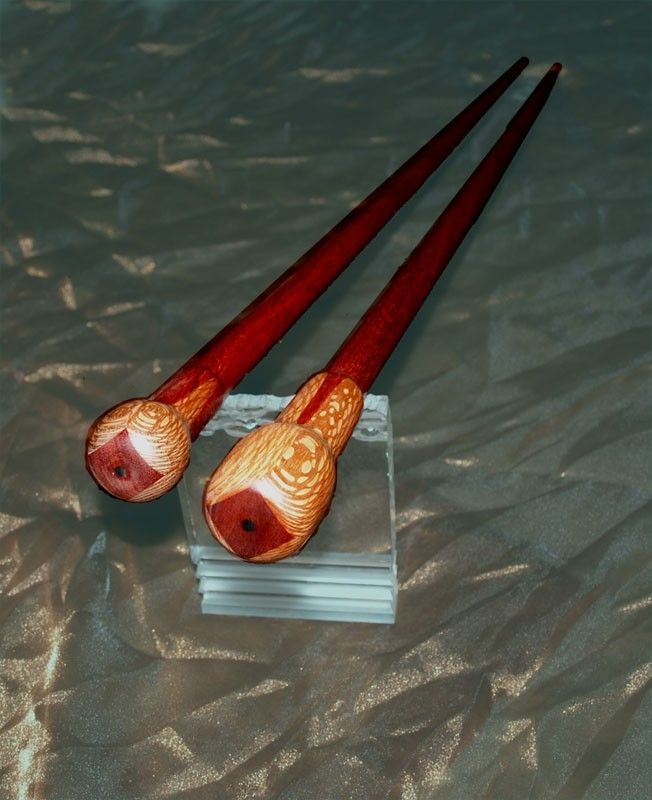This color photograph is taken indoors using artificial lighting and is in vertical portrait orientation. It captures two identically ornate wooden sticks, resembling drumsticks but more likely decorative or custom walking canes, given their intricate design. Both sticks taper to a red-painted end and feature a light wood grain handle on the opposite end. At the top, each stick has two knobs with a red square painted on the uppermost part. One knob appears circular, while the other is slightly more rectangular. These sticks rest on a stack of thick, clear plastic or glass squares, which enhances their decorative display. The scene is set on a heavily wrinkled gold-colored fabric, creating a textured background that emphasizes the fine details and craftsmanship of the wooden sticks.